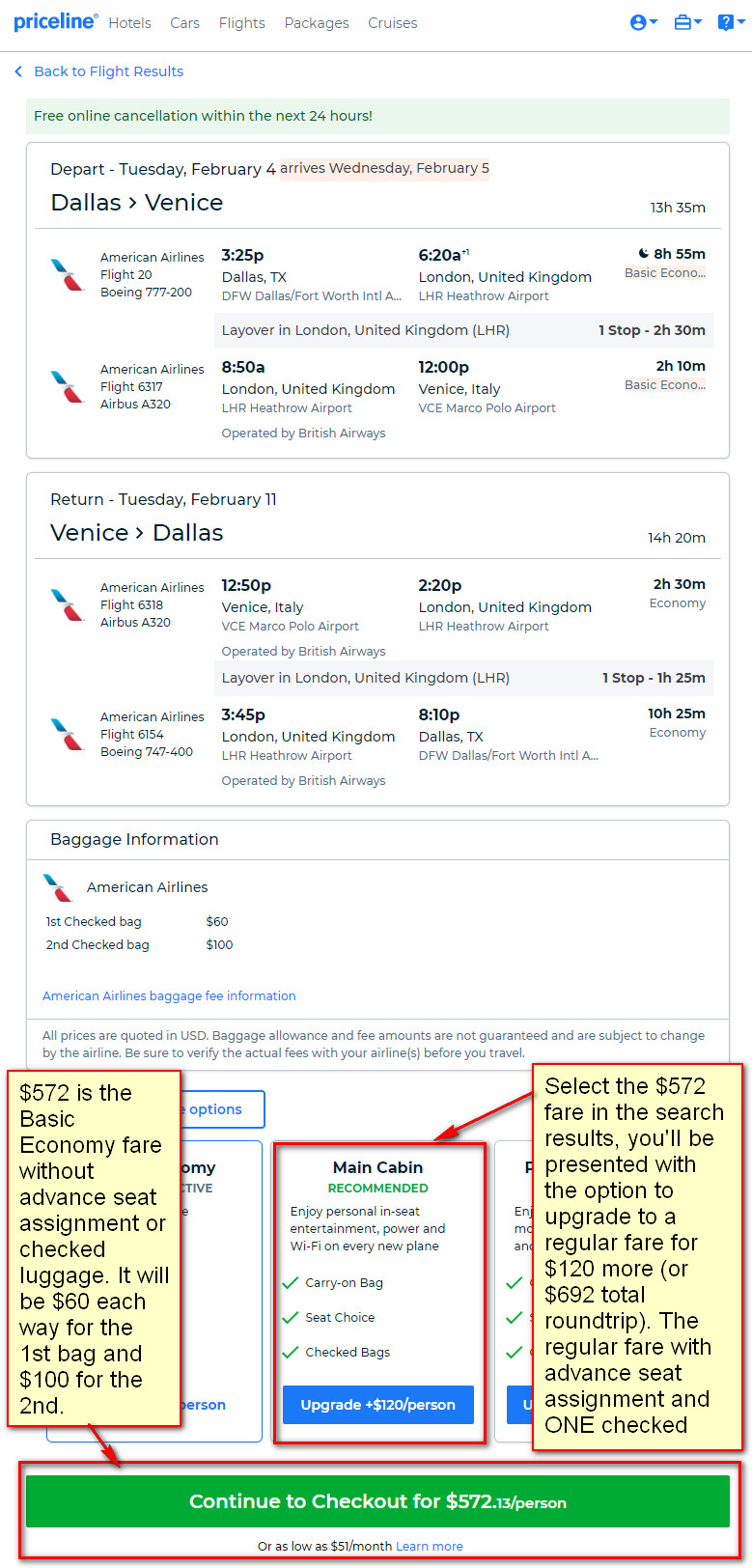The image displays a detailed summary of a travel booking on Priceline. In the upper left-hand corner, "Priceline" is highlighted in blue. Below, the options "Hotels," "Cars," "Flights," "Packages," and "Cruises" are listed in light black text. A notification states "Free online cancellation within the next 24 hours."

Travel details include:
- Departure: Tuesday, the 4th, from Dallas to Venice
- Arrival: Wednesday, the 5th, in Venice
- Return: Tuesday, the 11th, from Venice to Dallas

Baggage information for American Airlines is specified:
- Checked-in bag: $60
- Second checked-in bag: $100

The cost breakdown is provided for the basic economy fare:
- $572 for the basic economy fare without advanced seat assignment or checked luggage
- $60 each way for the first bag
- $100 for the second bag

The main cabin fare is marked as "Recommended," with an upgrade button available. The prompt indicates that selecting the $572 fare in the search results will present an option to upgrade to a regular fare:
- Regular fare: $120 more, totaling $692 for a round-trip
- Regular fare includes advanced seat assignments and one checked bag

The option to continue to checkout is provided, with the total fare amounting to $572.13 per person.